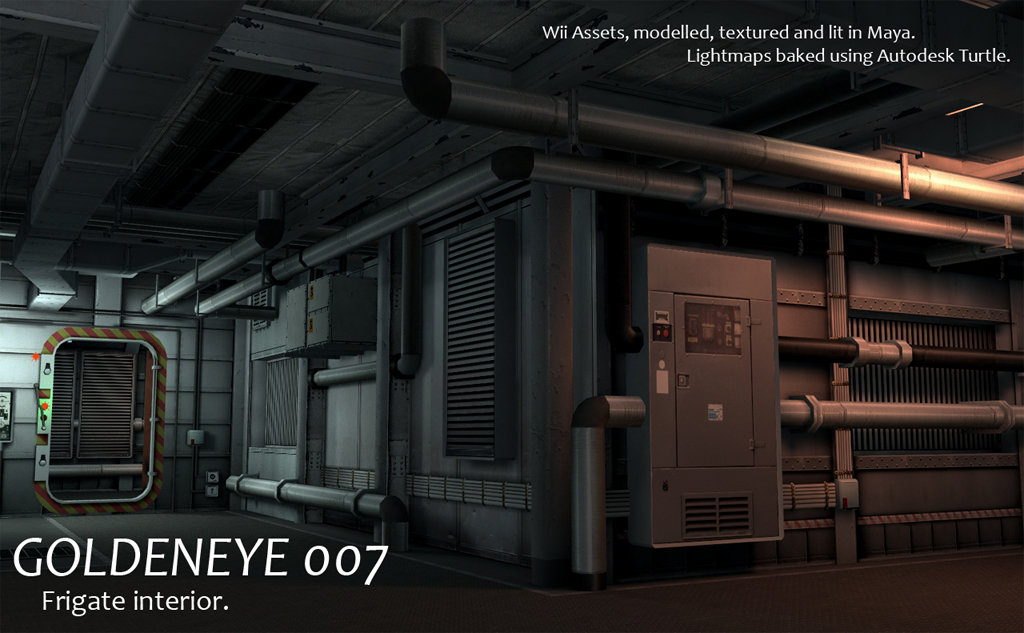This detailed image, likely a rendered illustration or screenshot from the video game GoldenEye 007, depicts the interior of a frigate. The bottom-left corner of the image is labeled "GoldenEye 007 Frigate Interior," while the top portion contains text that reads, "Wee Assets Modeled, Textured, and Lit in Maya. Lightmaps baked using Autodesk Turtle." The scene showcases a highly industrial, futuristic environment with a utilitarian aesthetic. Dominated by large metal pipes, vent conduits, and electrical conduits, this room resembles a factory or warehouse setting, possibly akin to an area in the basement of a business or hospital. An open door with red and yellow caution stripes is visible towards the left, accompanied by several metallic doors that look automated. The middle right features an electrical or utility box. The absence of people emphasizes the sterile, mechanical nature of the room, complete with high-tech red and green buttons on the left side of the image.